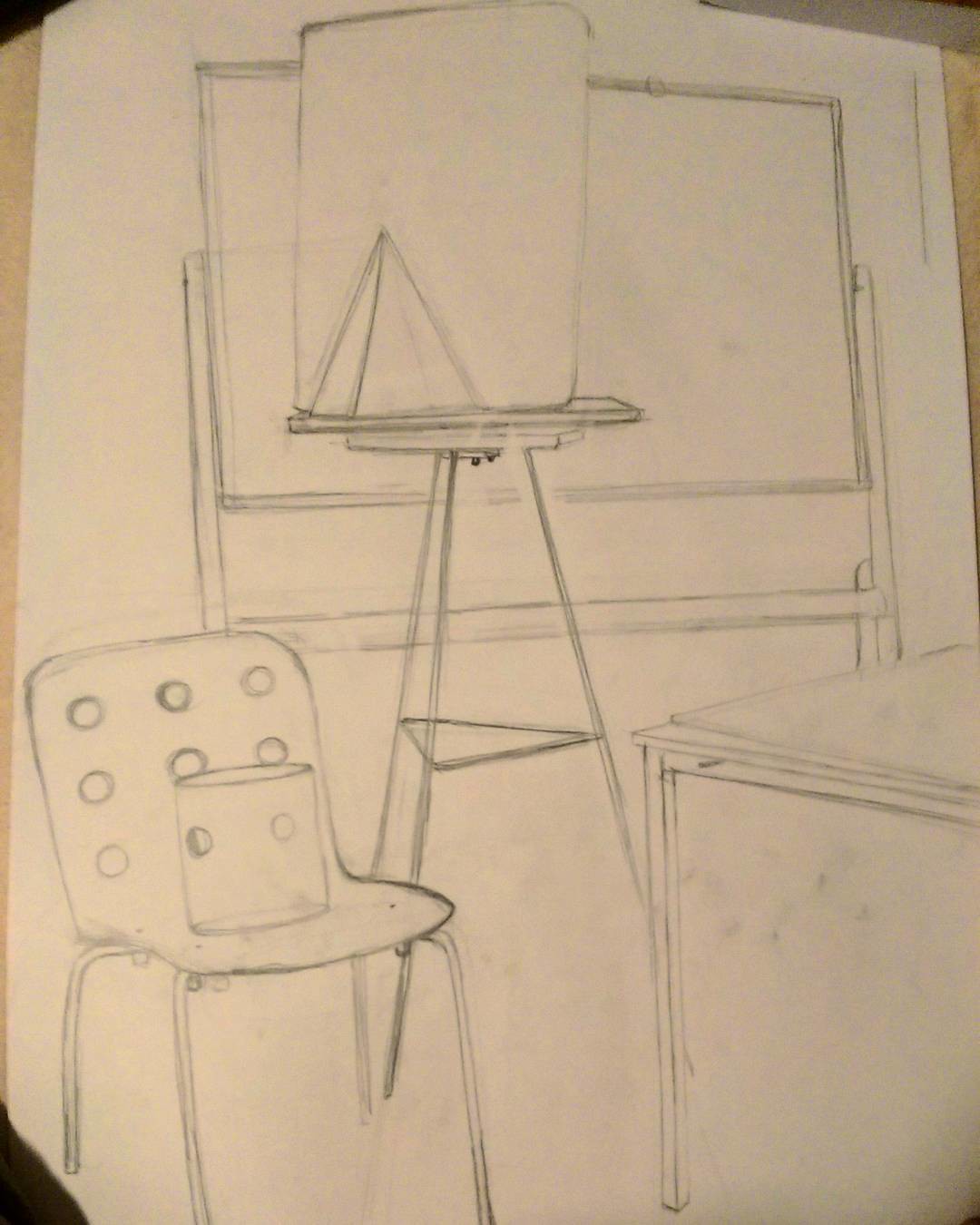In this detailed sketch, we observe a composition featuring a chair, a paint stand, and a chalkboard, all set against a light gray paper background with black areas in the very bottom left and top left corners. The chair, depicted from a front view, has a distinctive design with its backrest consisting of nine circular shapes, arranged in three rows of three. The chair's legs are notably thin, adding to its minimalistic appearance.

To the right of the chair stands a taller paint stand, topped with a square surface intended for a painting canvas. Positioned behind the paint stand is a square-shaped chalkboard with a frame that resembles a field goal post beneath it.

Additionally, on the right-hand side of the image, a series of lines implies the structure of a table. The entire drawing is rendered in shades of gray, blending seamlessly with the light gray sketching paper. In the upper right-hand corner, a slight tan hue adds a subtle contrast to the predominantly monochromatic artwork.